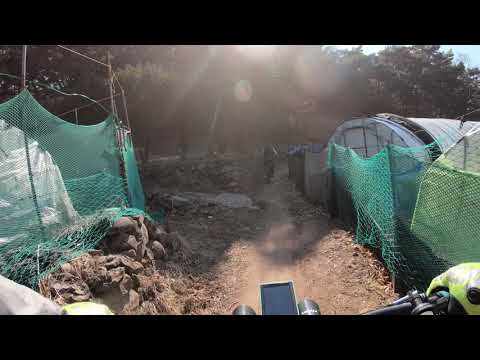The photograph captures an outdoor bike race held on a dusty dirt trail, bordered by dilapidated tents and green plastic netting of varying shades. The quality of the image is not optimal, appearing pixelated and marked by glare from the sun, which obscures the central top portion. The photograph features a rider's perspective, showing their yellow gloves gripping the handlebars of a dirt bike. Mounted on the handlebars are what appear to be lights and a cell phone. Ahead, another competitor is visible, adding to the sense of movement and competition. The background reveals tree cover and sunlight filtering through, which contributes to the overall brightness and reflects off the camera lens. The scene is framed by a black border on the top and bottom, providing a sense of confinement to the energetic activity within.